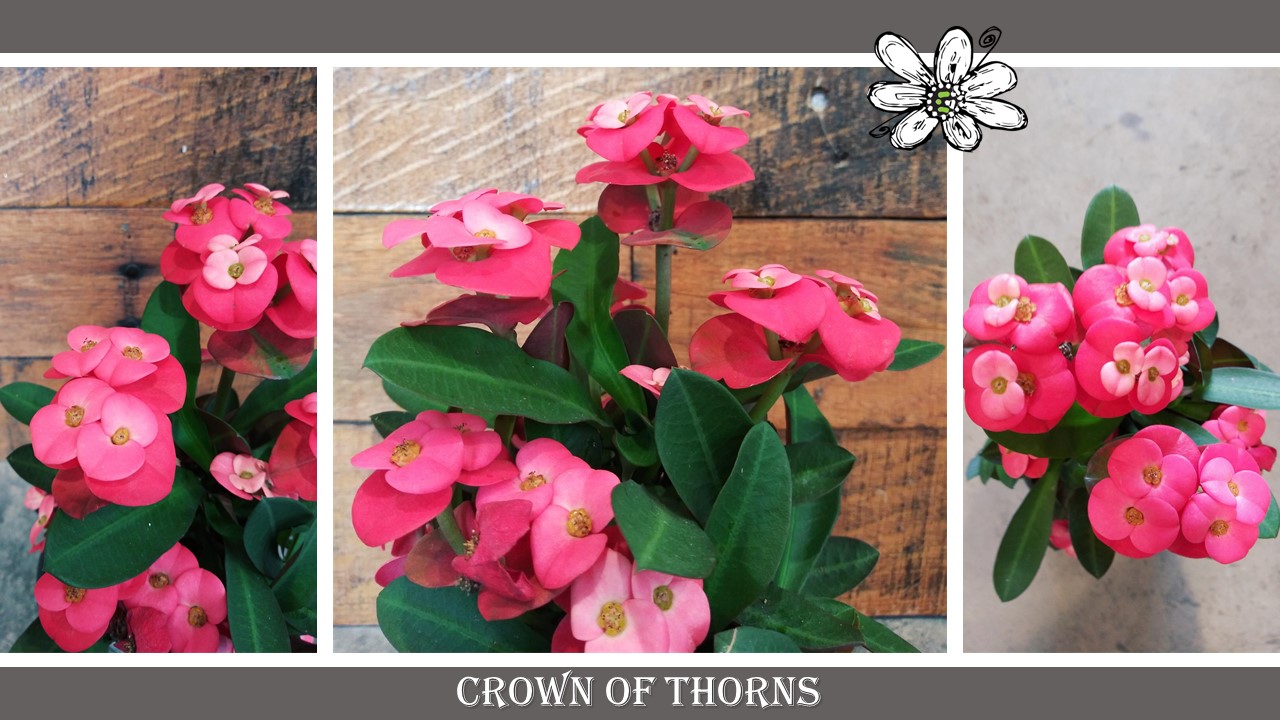The image is a collage specifically designed for online sharing, featuring three distinct photos of the same type of pink flower, known as the "Crown of Thorns," as indicated by the sharp white text at the bottom of the collage. The middle photo is larger compared to the two flanking images, creating a visually interesting composition. Both lateral images showcase the flowers against an old and weathered wooden background, while the central image displays them from an overhead angle on a marble table.

These flowers exhibit a striking combination of dark pink, light pink, and white hues, with small, flat petals that overlap each other, culminating in a dark yellow dot at the center. The oblong leaves with pointed tips add greenery to the scenes. A pencil sketch of a white daisy-like flower with a green center and tiny stems decorates the top of the collage, sitting between the second and third photos. This artistic element adds an extra layer of charm to the overall presentation. The entire arrangement is framed with gray borders on the top and bottom, unifying the composition.